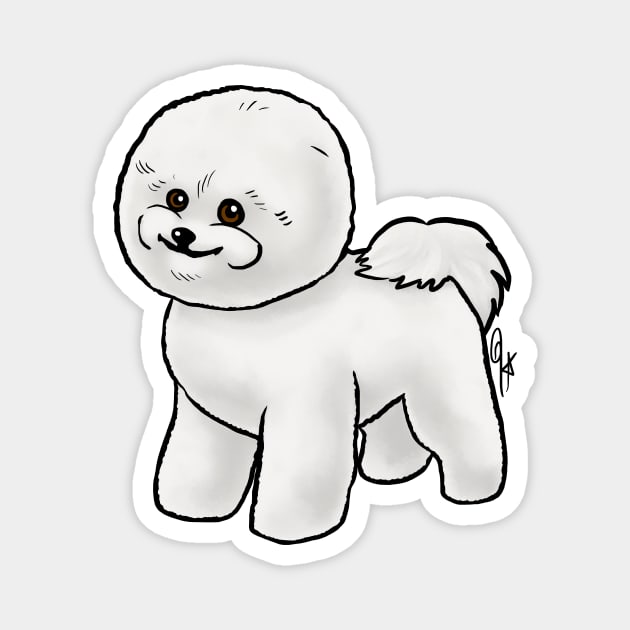The image is a detailed, hand-drawn sketch of a fluffy, white puppy with a rounded head and body, giving it a puffy appearance. The puppy is outlined in black ink on a white background, which is cut out as a sticker. It features expressive brown eyes, a black nose, and a smiling mouth, capturing a happy demeanor. Although the drawing lacks ears, the strokes indicating the fur suggest a young, playful dog, possibly a toy Pomeranian or a Maltipoo. The tail is particularly floofy, enhancing the adorable, puffy look of the dog. The background is gray, and there is a graffiti-style artist's signature at the base of the dog's tail. The simplicity and charm of the image make it suitable for a sticker that a teenager might put on their water bottle.